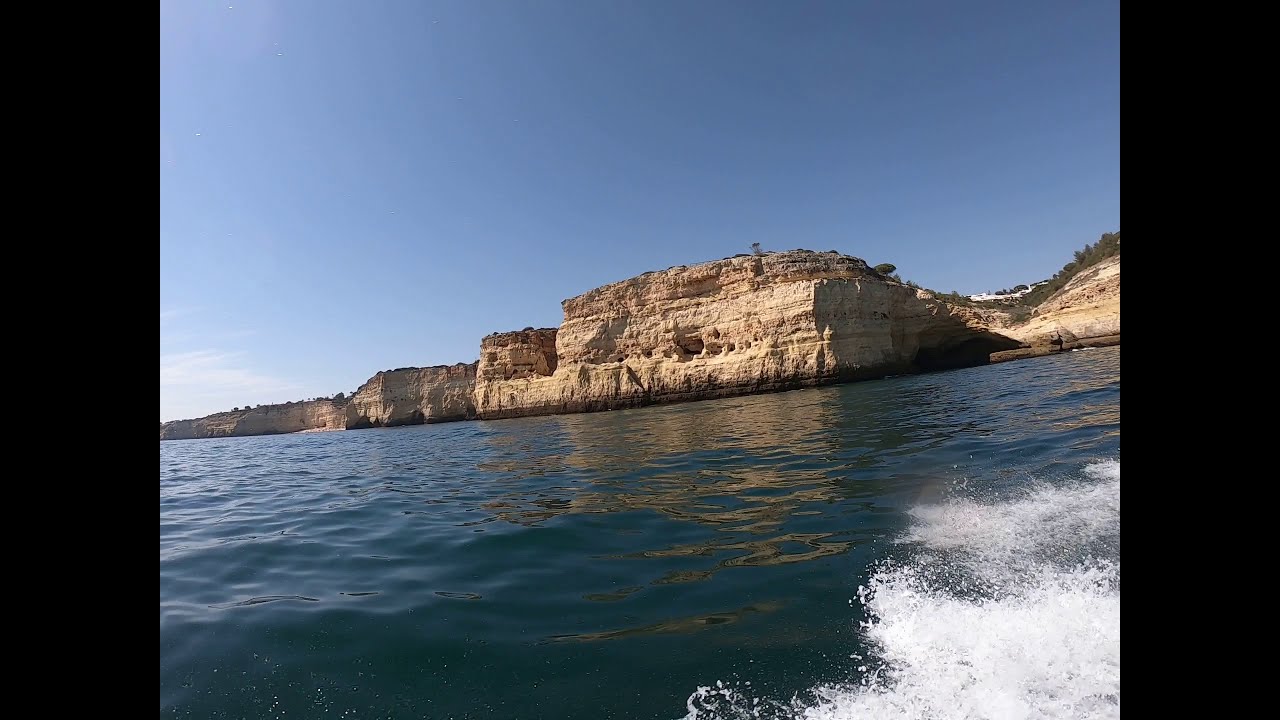This image captures a scenic outdoor setting from the perspective of being on a watercraft, such as a boat or jet ski. The frame is horizontally aligned with vertical black borders on both sides, giving the photo a square-like appearance within its boundaries. Dominating the middle of the picture are majestic cliffs that stretch from left to right, exhibiting a captivating range of light brown to dark brown hues. These cliffs are composed of whitish brown clay and appear to have been cut off sharply, indicating their impressive height and ruggedness.

Below this formidable cliffside lies the expansive body of water, characterized by a deep blue turquoise shade that transitions to a more bluish-gray tone. The water near the front of the image shows turbulent white motion, suggesting the splash and wake of the moving watercraft. Above, the sky is a bright, clear blue with a few feathery white clouds positioned toward the left side of the image, adding a touch of serenity to the overall scene. This richly detailed landscape conveys both a sense of adventure and natural beauty, with the contrasting textures and colors of the cliffs, water, and sky coming together harmoniously.